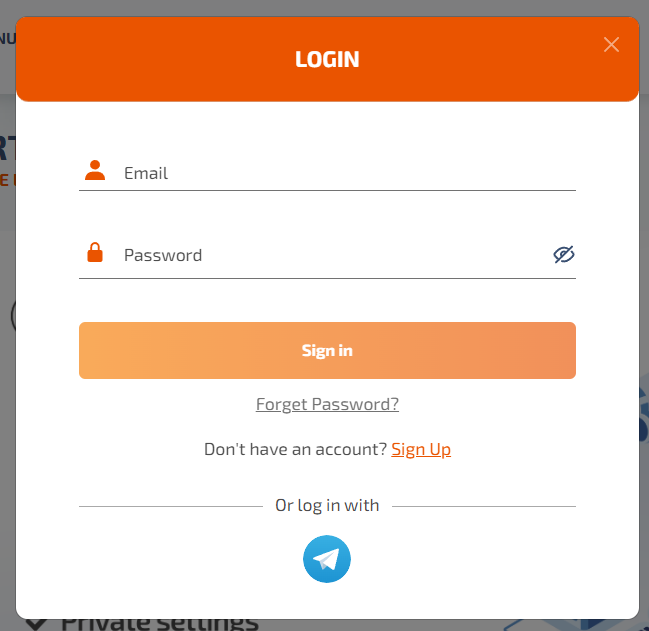The image depicts a login pop-up window from an unspecified website or application. The background of the login area is white, while the broader backdrop contains indistinct text that does not reveal the identity of the webpage or app. At the very top of the window, there's an orange bar with the word "Login" written in white.

Below this bar, the window includes fields for "Email" and "Password," each accompanied by small orange icons—a mail envelope for the email field and a lock for the password field. The password field also features an icon of an eye with a diagonal slash through it, indicating that the typed password will be obscured by dots to ensure privacy.

There's a light orange button for submitting the login information. Beneath the password field, there is a hyperlink labeled "Forgot Password?" for users who need to recover their credentials. Further down, a prompt reads "Don't have an account? Sign up," with "Sign up" highlighted in orange and acting as a clickable link.

Finally, the window provides an alternative login option, stating "or login with," followed by an icon resembling the logo of the Telegram app.